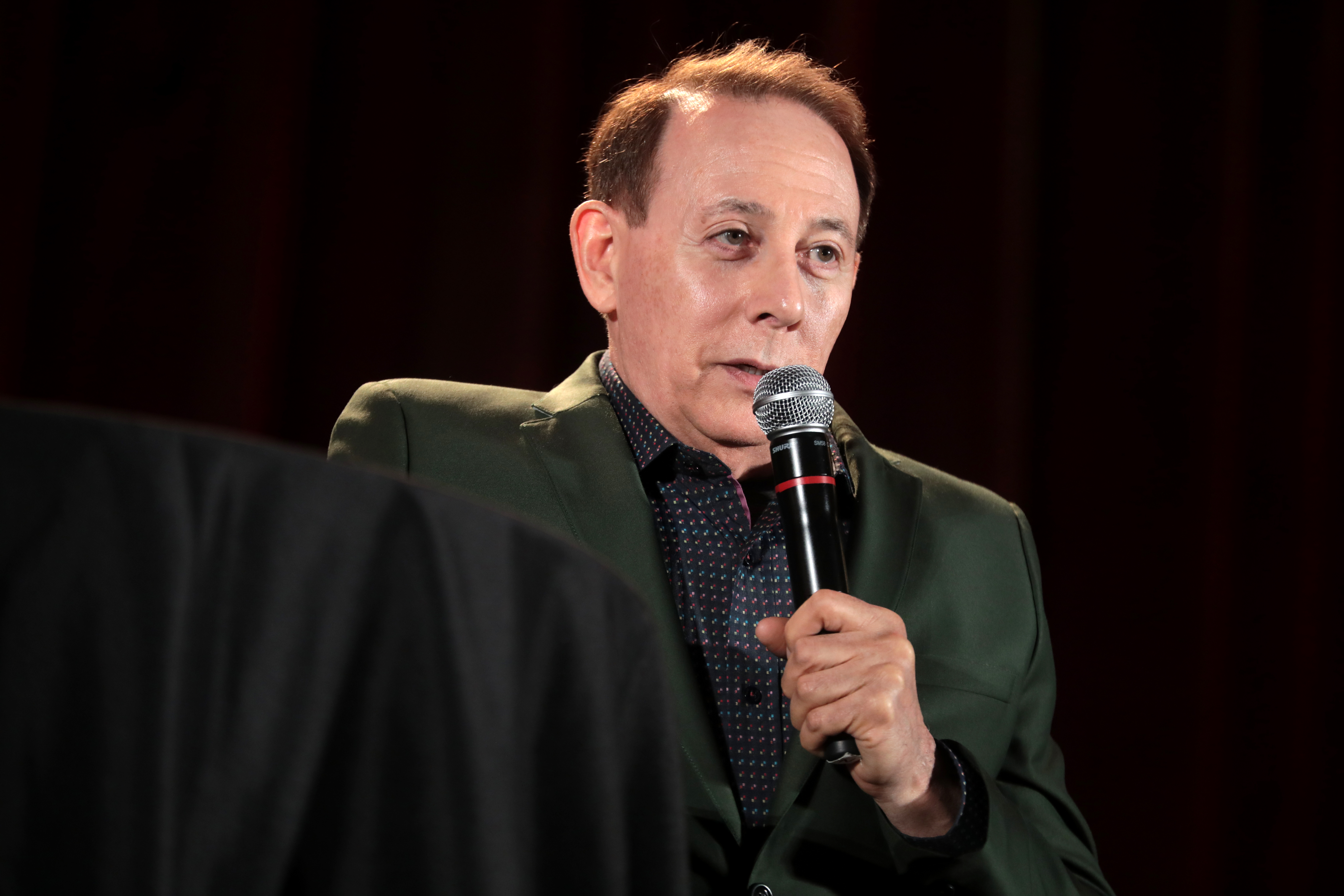The image features a man, likely in his 60s, who has fair skin and brownish-red hair parted on the side, holding a microphone with his left hand. He is wearing a forest green sports jacket over a black collared button-down shirt adorned with small colored dots. The man is positioned at an angle, facing from the left to the right, and his gaze is directed slightly forward and down. The background is entirely black, adding a contrast that highlights his figure. In the lower part of the image, there appears to be a table with a black tablecloth. The microphone, held in his left hand and positioned near his mouth, is black with red and gray accents. The setting suggests that the man is engaged in giving a speech or talk.